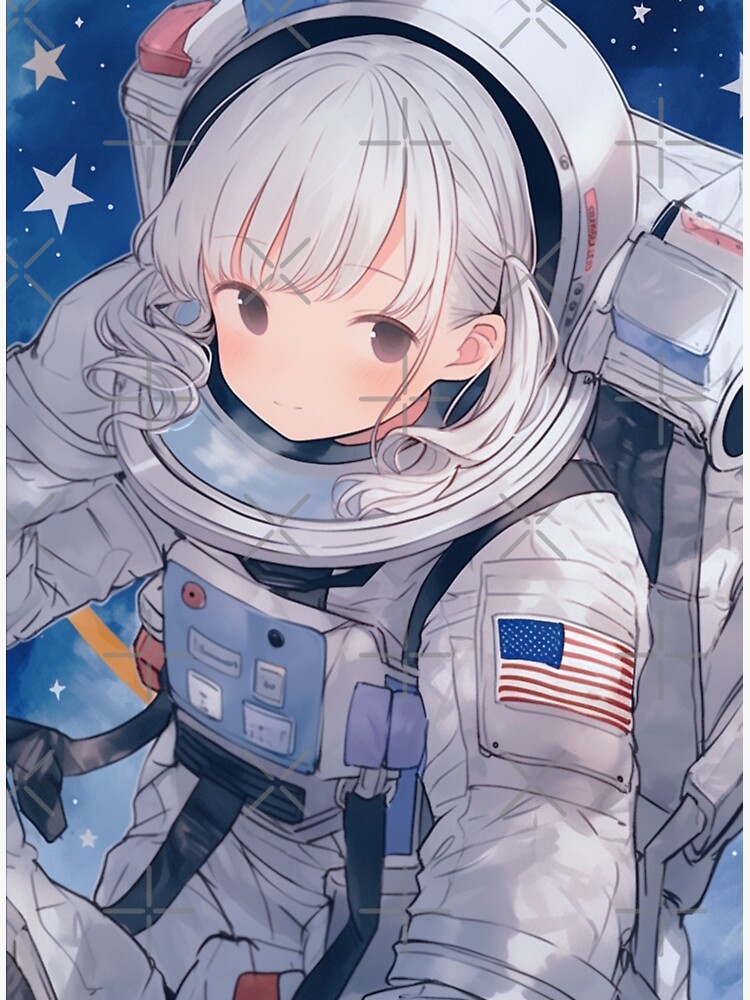This image showcases a highly detailed, anime-style drawing of a young girl in an astronaut suit, set against the vastness of space. The girl is positioned at the center of the image, captured in a dynamic pose with her left hand outstretched forward. Her suit is predominantly shades of gray and white, with the sunlight creating varying lighter and darker tones. Notably, the American flag is visible on her left shoulder, adding a patriotic touch to her attire.

Her helmet is white with subtle red and blue accents, complementing the colors of the flag. The suit features a chest device adorned with numerous buttons and a backpack secured by black straps. Although she doesn't have a nose or an overt smile, her expression is soft with a faint smile, and her enormous, glistening eyes — characterized by dark pupils and white sclera — gaze upward. Her hair is styled in ponytails and is a striking grayish-white, enhancing her youthful and otherworldly appearance.

The background is a dark, star-filled sky, where the stars are whimsically illustrated as five-pointed shapes. The colors in the picture range from deep blues and blacks to pale blues, purples, and oranges, creating a serene yet vibrant cosmic scene. Overall, the artwork beautifully amalgamates the charm of anime with a space exploration theme.